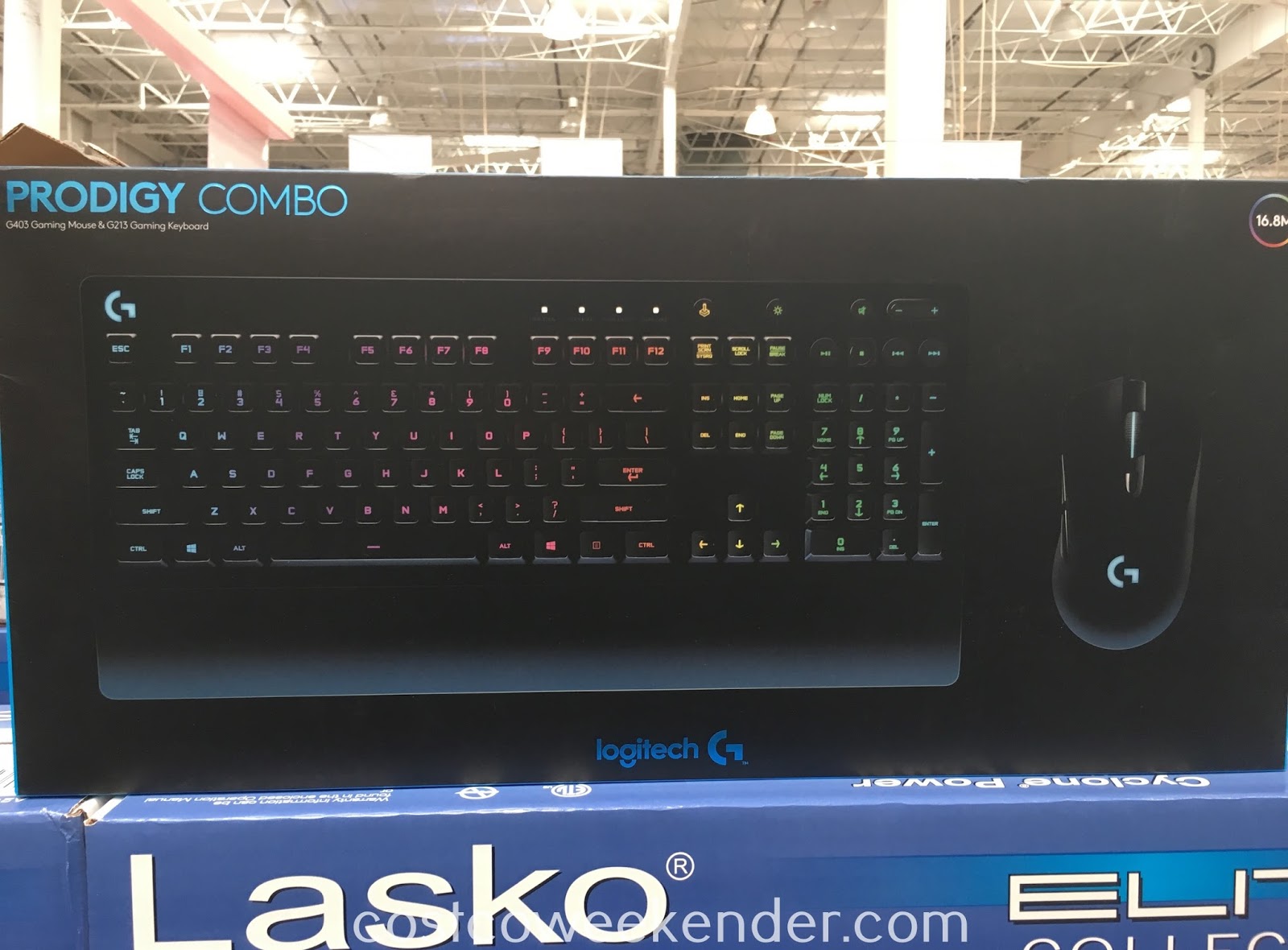The top portion of the image showcases the interior of a warehouse, specifically focusing on the white roof and rafters. Positioned slightly left of center is a light that is turned on, whereas to the right of it, there are three lights, all turned off. Approximately two inches from the right edge, a column descends, mirrored on the left side by another column. The backdrop from this point downwards to about two inches from the bottom is solid black.

In the center of the frame lies a stylish keyboard, illuminated by a variety of colors - red, yellow, green, and pink - on the number keys, contrasting against its black body. The keyboard is part of a boxed set, revealed in the narrative text overlay.

The top left corner of the box features the bold, all-capitalized text "PRODIGY COMBO" in blue. Below this, in white lettering, are the words "G403 Gaming Mouse and G213 Gaming Keyboard." A small outlined circle on the left side, with a black center, indicates "16.8". Adjacent to this is an image of a black mouse branded with a blue letter "G" symbol that resembles a stylized "C."

Across the bottom of the box, "Logitech" is written in blue with a distinctive 'C'. A hint of another blue box can be seen below this, with the white, bold text "Alaska" in the left corner. On the right side is the partial text "ELI," which trails off the edge of the image.

Additionally, there is a watermark at the bottom that reads "CostOfWeekender.com" in black or light blue text.